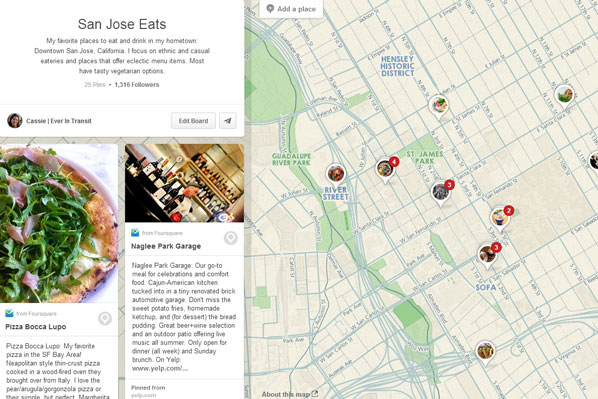The website "San Jose Eats" is a comprehensive guide focusing on ethnic and casual eateries in downtown San Jose, California. On the left side of the homepage, there is a section titled "My Favorite Places to Eat and Drink in My Hometown." This section highlights the website's emphasis on unique menu items and restaurants offering tasty vegetarian options.

The webpage features a beautiful image of a dish named "Pizza Bacalupo," presented by a contributor named Cassie. Cassie's profile is shown, indicating she is a white person. Her profile also includes the status "Ever in Transit." One of the highlighted eateries is called "Naglee Park Garage," and the website showcases an interior image of this restaurant. The photograph includes a view of the bar area, complete with a bartender and an array of wine bottles, emphasizing the inviting atmosphere.

In one of the central sections, a large map with numerous pins illustrates the locations of various restaurants within the historic district and surrounding areas. This map provides users with a visual guide to explore where these eateries are situated.

The profile indicates that "San Jose Eats" has 1,316 followers and numerous posts (the precise number appears to be 25 or 23). This website serves as a detailed and visually engaging resource for food enthusiasts looking to explore the culinary delights of downtown San Jose.